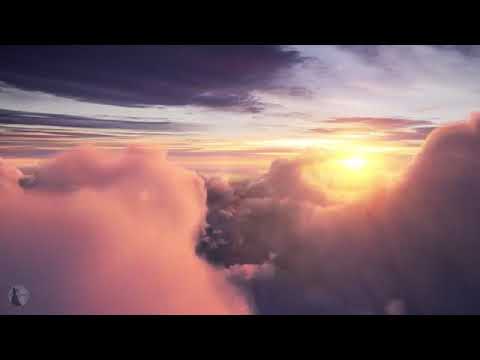This photograph, likely taken from an airplane, captures a spectacular sky at either sunrise or sunset. The viewer is positioned high up, surrounded by a mixture of thick, fluffy clouds below and ominous, dark gray and purple storm clouds above. The Sun, a brilliant yellow orb, is nestled between these layers of clouds, casting a golden glow that radiates outward. Below the Sun, the sky is a gradient of deeper hues transitioning from shadowy to light. Far above, patches of darker clouds are interspersed with glimpses of blue. The bottom left of the image contains a barely visible circular icon with an indistinguishable shape inside. The scene is one of contrast and awe, showcasing the serene and turbulent elements of the sky from an enthralling aerial perspective.